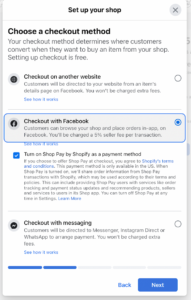**Detailed Image Description:**

The image appears to be a screenshot taken from a digital device, likely a laptop or smartphone. It primarily consists of a prominent white box that contains various sections of text. Some portions of the text are blurry and difficult to read, especially those that are smaller in size.

At the top center of the white box, there is a bold title in black text that reads, "Set up your shop." To the right of this title, there is a small circular icon with an "X" inside it, functioning as a close button.

Below the main title, the following line of black text states, "Choose a checkout method." The next line elaborates with a brief description: "Your checkout method determines where customers convert when they want to buy an item from your shop. Setting up checkout is free."

Further down, there is a bullet point (depicted as a black circle) followed by the option "Check out on another website." Under this option, there are two lines of gray text that are too small and blurry to decipher, along with a line of blue text that is also hard to read.

The next section features a Facebook icon on the left, adjacent to black text that states, "Check out with Facebook." This option seems to be active, as indicated by a blue checkmark inside a blue circle on the right side. This entire section is enclosed within a gray box.

Following this, there is a blue checkmark next to the text, "Turn on shop pay by Shopify as a payment method." There is an additional paragraph of text in black and blue, but it is too small and unclear to read.

Continuing down, another bar features the Facebook Messenger icon on the left and black text that reads, "Check out with messaging." This section includes a sentence of gray text that is similarly difficult to read due to its size and blurriness.

At the very bottom of the white box, there are two blue bars out of five, indicating that the user is currently on page 2 of 5. The remaining three bars are not highlighted. Below this progress indicator, there are two navigation options in blue text: "Back" on the left and a blue square with the word "Next" inside it on the right.